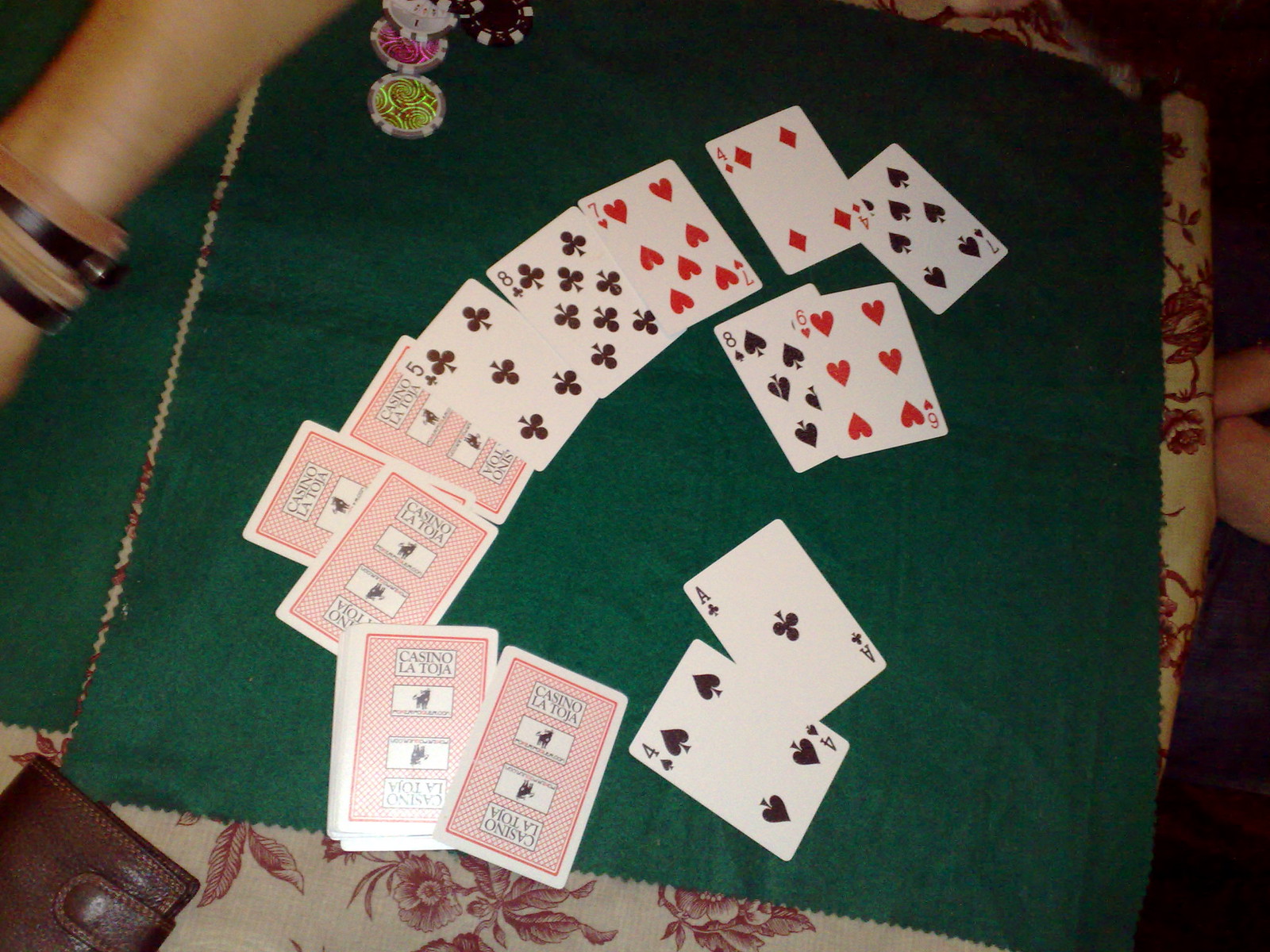The image captures a vibrant scene of a tabletop adorned with playing cards and poker chips. The table is covered with a beige tablecloth patterned with red flowers, adding a touch of elegance. On top of this, there's a green cloth spread out, serving as a makeshift playing surface. Scattered around are several playing cards, both face up and face down. Visible face-up cards include a 5, an 8, a 7 of hearts, a 4 of diamonds, a 7 of hearts once more, and an 8 and a 6 placed next to each other. Additionally, there's an ace and a 4 of hearts slightly separated from the main group. Many cards lie face down, displaying a 'Casino La Toho' design on their backs, characterized by a red checkered pattern with four white images and a white border. At the top of the green cloth are poker chips of various colors, including black, green, brown, and violet. A hand partially enters the frame from the top, though largely out of view, suggesting the presence of players engrossed in their game.